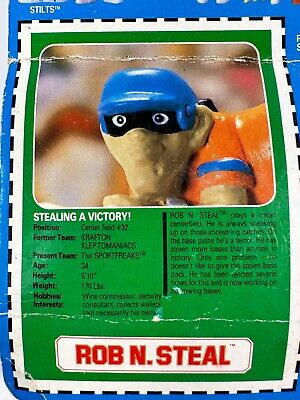The image depicts an aged, colorfully illustrated baseball card featuring a wax figure of a cartoon baseball player. The card itself is portrait-oriented with a blue background and a black broken line border, showing signs of wear with wrinkle marks across the top and bottom. The central focus is a photograph of the wax figure, occupying the top half of the card. The figure wears a blue helmet and a black face mask that obscures its facial features, with only an ear partially visible. It appears to be crouched forward, extending its body to the right, dressed in a red jersey with a blue stripe on the sleeve and orange gloves, possibly batting gloves. This photograph is set within a green vertical rectangle.

Below the photograph, the card caption reads "STEALING A VICTORY" in white text, accompanied by two columns of black text detailing the player’s position as center field, number 32, and mentioning former teams, including Krafton. The bottom of the card features a white horizontal rectangle with red text in all caps that reads "ROB END STEAL." The design blends photographic representationalism with graphic elements, creating a playful yet nostalgic aesthetic, hinting that the card is a collectible item targeted at children.